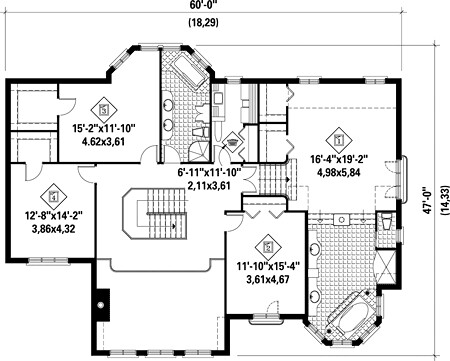This detailed schematic illustrates the floor plan of a building, rendered in black markings on a white background. The layout clearly denotes a single floor, yet the presence of a central staircase hints at additional levels above or below. The dimensions of the building are provided: 60 feet in width and 47 feet in length.

The entrance is positioned on the right side of the blueprint, featuring double doors that open into a spacious main room. The schematic meticulously details the dimensions of each room, with the main room measuring 16 feet 4 inches by 19 feet 2 inches. Notably, the design includes a large bathroom, but no bedrooms are indicated. Each room's specific dimensions are clearly labeled, providing a comprehensive overview of the interior layout. Stairs suggest further exploration is possible beyond this single floor plan.